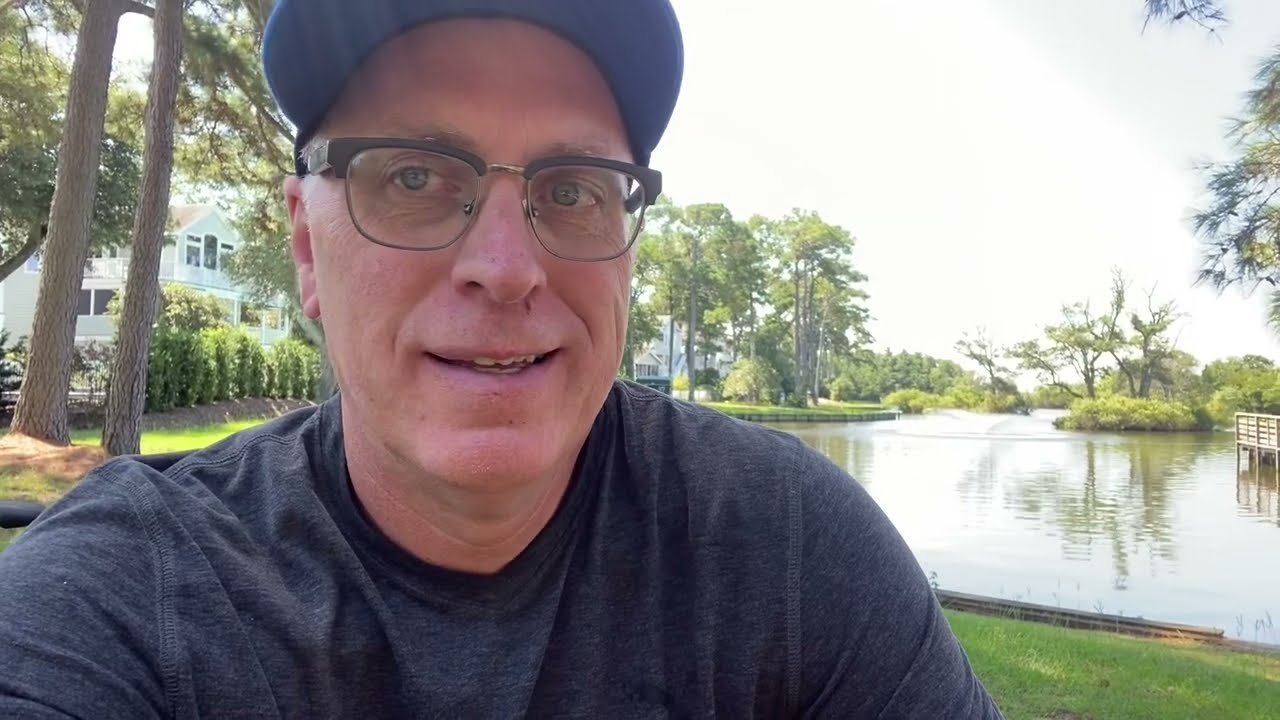This image captures a slightly older white man, perhaps in his 40s, taking a selfie. He is wearing a dark gray t-shirt and a blue baseball cap with a black brim. His glasses have thick black frames at the top, separated by a gold bar at the nose bridge. He has either blue or green eyes, which are noticeable through his glasses. The man is smiling slightly, showing a bit of his teeth.

In the background, there is a serene pond with a glossy surface reflecting the surrounding greenery, which includes tall trees, shrubs, and grassy banks. To the right, there is a wooden dock or boardwalk extending out over the water, suggesting a residential area with backyards that reach out to the pond, creating a picturesque and tranquil backyard scene. The bright, lush foliage and overall setting indicate it is summertime.